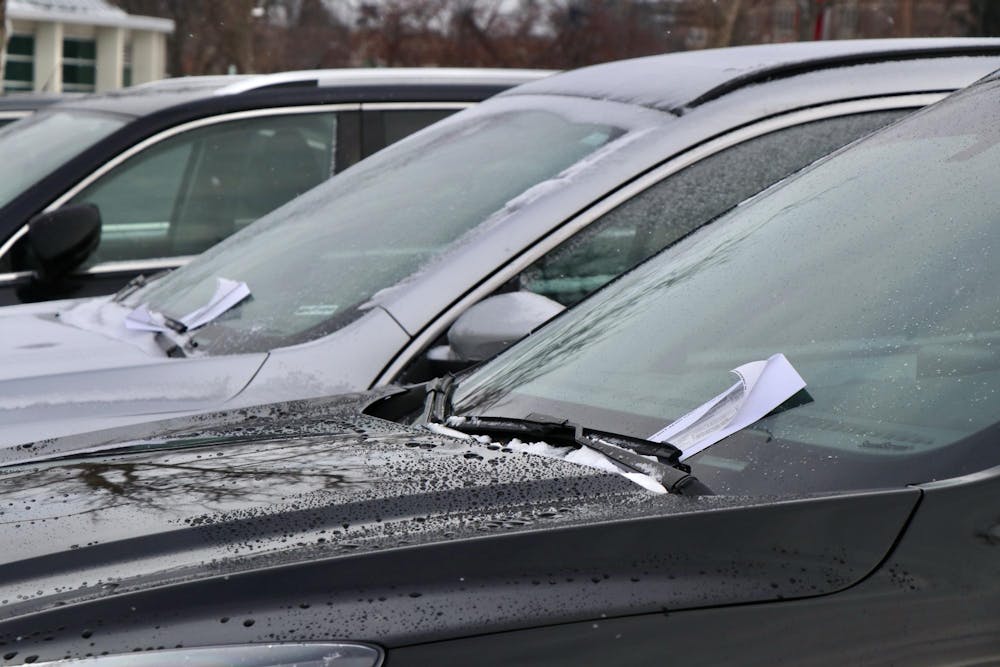This photograph captures a somewhat close-up view of three cars lined up side by side, partially obscured by darkness. The first car in the foreground is black, with fresh raindrops speckling its hood and windshield. A piece of white paper, possibly a ticket, is tucked under its windshield wiper. The middle car is silver, also sporting a noticeable piece of paper under its windshield wiper, and appears wet from recent precipitation, perhaps rain or snow. The third car, barely visible, is another black vehicle. All three cars are parked against a backdrop of dimly-lit trees, suggesting a winter setting. In the distance to the left, a white building is discernible, further adding context to the cold, dark ambiance of the scene.